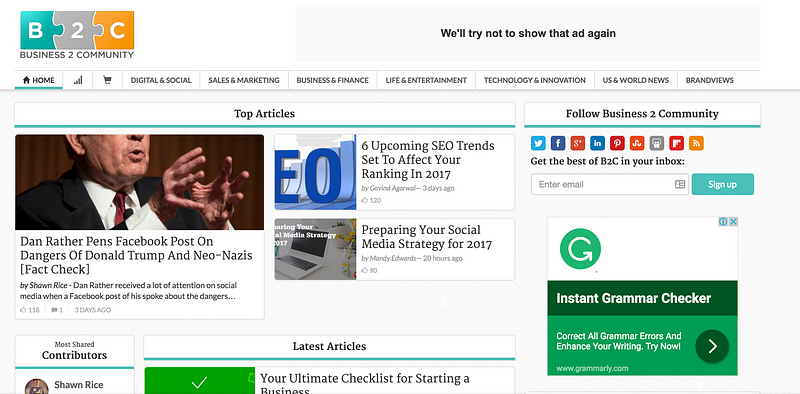Screenshot of the Business to Community website featuring a well-organized layout with several tabs and categories for easy navigation, including Home, Digital & Social, Sales & Marketing, Business & Finance, Life & Entertainment, Technology & Innovation, U.S. & World News, Brand Views, Top Articles, and Follow Business to Community. Prominent headlines include "Dan Rather's Pin about a Facebook Post on the Dangers of Donald Trump and Neo-Nazis, Fact-Checked," "Six Upcoming SEO Trends Set to Affect Your Ranking in 2017," and "Preparing Your Social Media Strategy for 2017." The site invites users to subscribe for updates with a prompt to enter their email in the "Get the Best of BTC in Your Inbox" section followed by a sign-up option. Additionally, a green and dark green ad for an "Instant Grammar Checker" tool, which promises to correct all grammar errors and enhance your writing, is prominently displayed. The "Most Shared Contributors" section highlights Sean Rice, and recent articles include "Your Ultimate Checklist for Starting a Business." All content is set against a clean, white background, while the ad features a greenish backdrop.